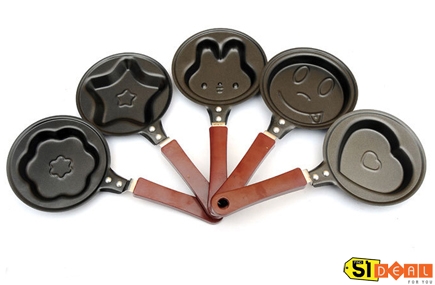The image depicts a set of five kid-friendly pancake or cookie molds, each featuring a distinct and charming shape. These molds consist of small, cast iron-like metal skillets attached to brown wooden handles, providing a classic, rustic look. The handles are described as brown in one account and red in another, indicating they may have wooden accents or a mix of red and brown. The set includes molds shaped like a flower, star, bunny (possibly Miffy), smiley face with a tongue sticking out, and a heart within a heart. The molds are designed to be practical and versatile, ideal for making pancakes, cookies, or even playful activities using materials like Play-Doh. The bottom right corner of the image features a yellow price tag displaying "5-1" and an orange square background behind white letters spelling "DEAL," with the phrase "for you" written underneath. These cute, themed molds are perfect for creating special treats for various occasions like Valentine's Day or Easter, engaging children in fun cooking or crafting projects.